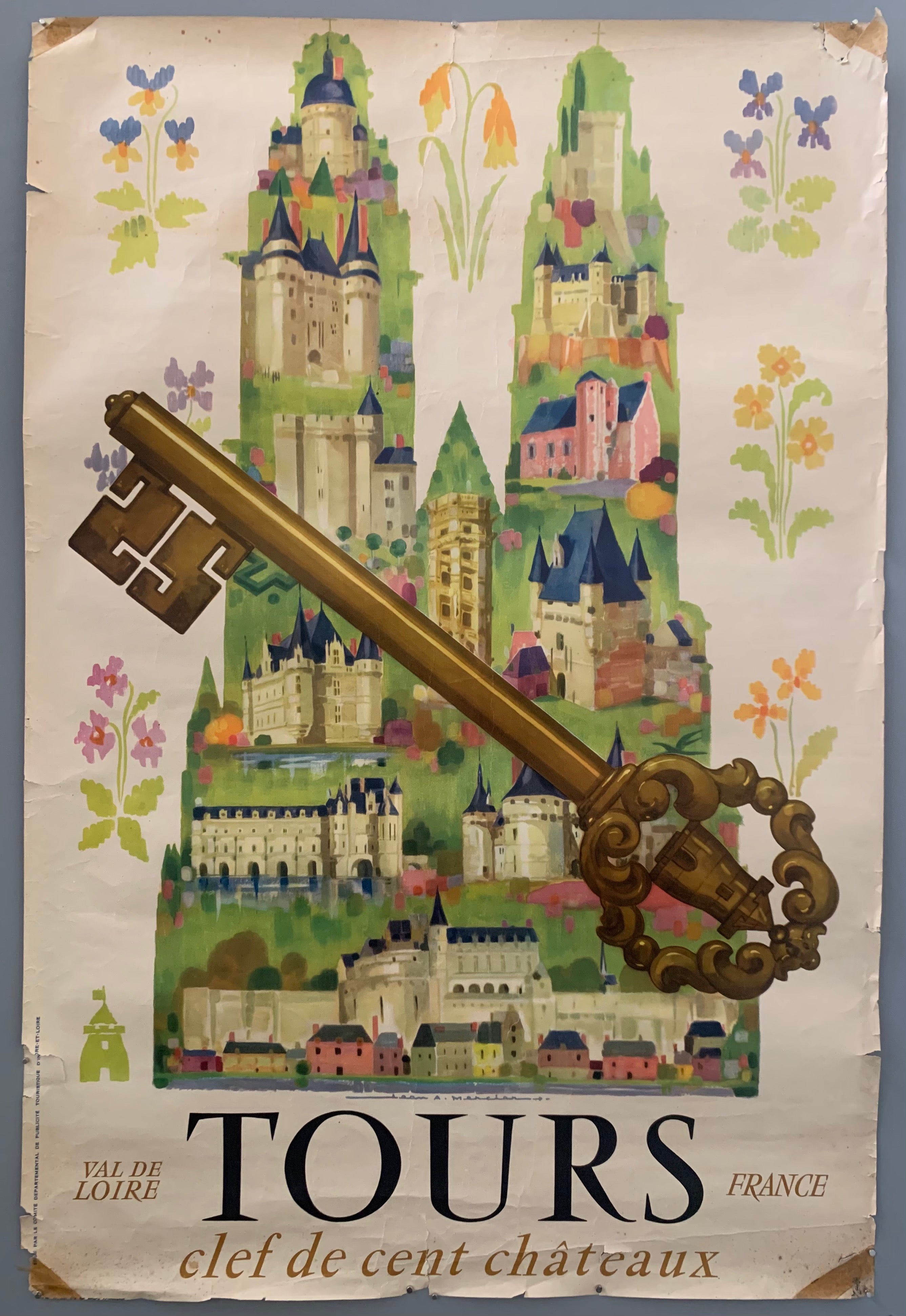This image is a detailed advertisement for a tour company in France, specifically promoting the Val d'Or Tours in the Vallee des Seigneurs (Valley of the Lords). At the center of the illustration is a large brass skeleton key adorned with intricate filigree, which contains a small house within a circle. This key overlays a prominent silhouette of a green castle, within which several vividly illustrated castles of varying sizes and designs are arranged. Most of the castles are depicted in white with blue peaked roofs, although some variations include a pink castle with a blue roof. Below this central motif, regular houses can be seen in front of a larger castle. The background and edges of the page are white with dark brown corners, and the entire page rests on a gray surface. Surrounding the green castle silhouette are colorful flowers in blue, purple, yellow, pink, and green, adding a vibrant touch to the composition. Text is interspersed throughout the image: "Val d'Or Tours France" and "Clé de Saint Château" are prominent, with "Tours" labeled beneath the castle silhouette and "France" to the right. Additional words in French are also visible near the left side of the silhouette.